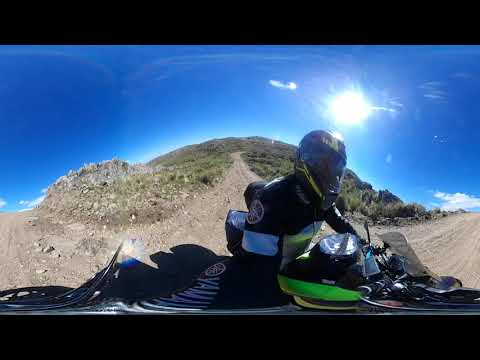A motorcyclist takes a dynamic selfie while riding a green and black Yamaha motorcycle on a tan dirt and gravel path. Their black, full-face helmet, adorned with yellow words and a dark visor, complements their black long-sleeve leather jacket, which features silver bands and a red circular logo on the arm. The bike sports a dark colored see-through windscreen. The setting is outdoors under a bright, rich blue sky with very few white clouds, and the sun shining overhead. Sparse, dry-looking green vegetation lines both sides of the well-used path, highlighted by multiple tire tracks. The photo, taken with a selfie stick or similar device, captures the energy of a sunny day adventure amidst rugged terrain.